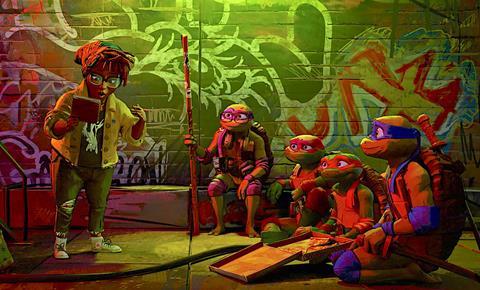In a detailed screenshot from the recently released Teenage Mutant Ninja Turtles animated movie, a young Black woman with dreads, glasses, and a yellow jacket over a t-shirt, is engrossed in speaking to the four Ninja Turtle brothers. She holds a notepad the size of her head in her right hand, possibly discussing important details or solving a mystery. They're situated in an alleyway, suggested by the graffiti-covered brick wall in the background, reminiscent of New York City's typical street art. The turtles, drawn in detailed 3D animation, display their unique characteristics: Donatello in purple with a staff and glasses, Raphael in red, Michelangelo in orange holding a pizza box, and Leonardo in blue with two katanas. Each turtle listens attentively to the woman, indicating their deep interest in what she is saying. The scene captures a vibrant mix of action and camaraderie, fully immersing viewers in the turtles' world.